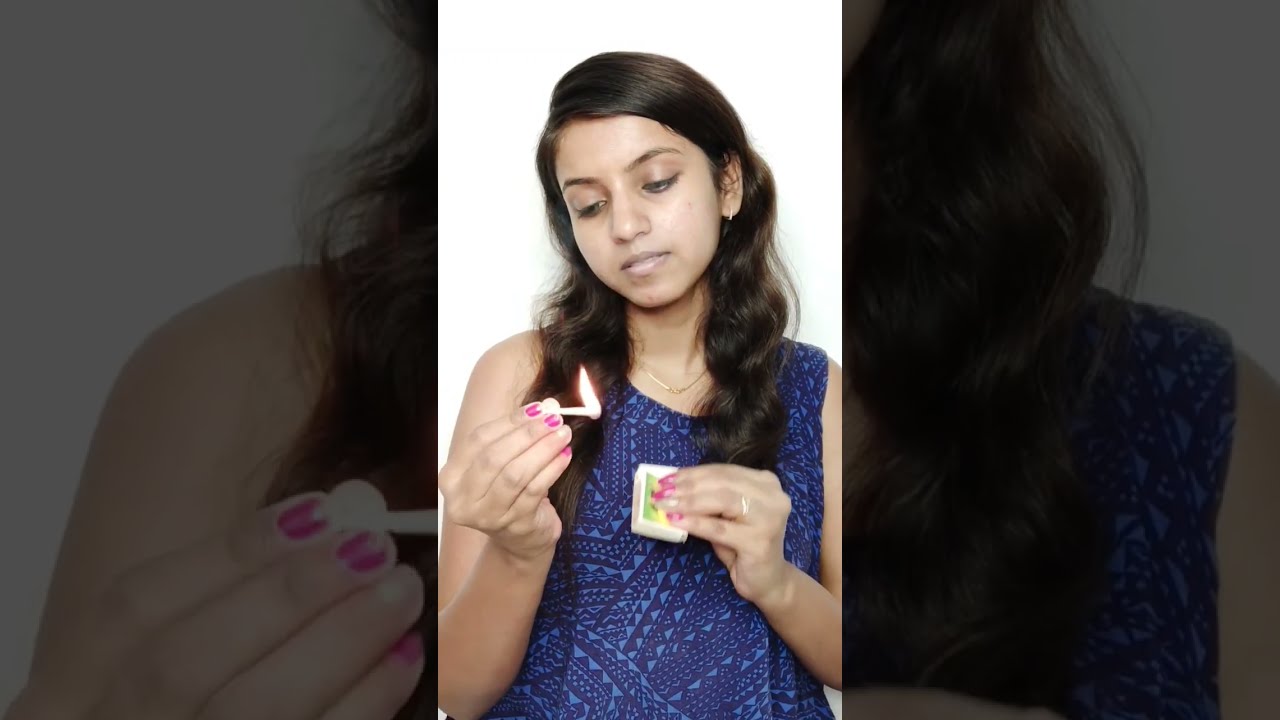In the image, a girl with long brown hair, that she has tucked behind her ears, is central to the white background. She is wearing a blue tank top adorned with light blue triangles and dotted line patterns. Her left hand holds a lit match, while her right hand holds a matchbook. The flame from the match illuminates her face as she gazes downward at it, displaying her pink-painted fingernails. On either side of her are two rectangular, zoomed-in versions of the same image, darkened and faint, showcasing parts of her hair, shoulder, shirt, and fingers. The girl's complexion has a slight tan, and her hair flows wavy down to the sides of her chest.